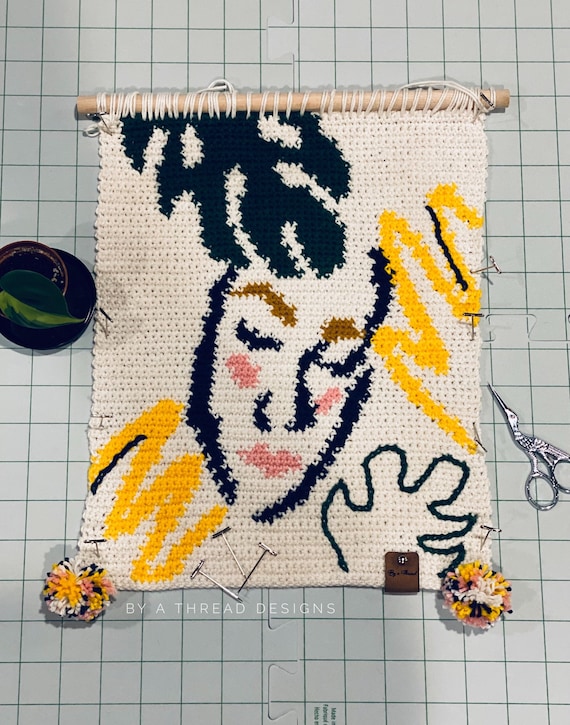The image features a crafting scene, likely from a book or an Etsy page, displayed on a white or grey surface with a grid pattern of green or blue lines, resembling graph paper. Centrally, there is a decorative crochet or stitching project on an off-white fabric square, featuring a detailed line drawing of a woman's face with black hair, brown eyebrows, closed eyes, pink cheeks, pink lips, and yellow squiggles around her shoulders and head. This artwork is tied to a dowel and adorned with two pom poms at the bottom, colored pink, navy blue, yellow, and white. On the lower part of the fabric, three long pins are resting, and a brown leather square is attached. The right side of the image shows a small pair of silver scissors designed to resemble a bird. A small potted plant with one visible green leaf is partly visible on the left side of the image. At the bottom of the scene, the text "By A Thread Designs" is prominently displayed in white capital letters.